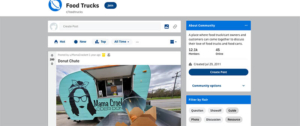This screenshot captures a portion of a website with suboptimal quality, making the text difficult to read. The layout features a rectangle shape, with the background transitioning from medium to light gray on the left and right sides to white at the very top. The top section prominently displays the title "Feed Tracks" alongside its logo, positioned on the left. The logo consists of a blue circle containing a white schematic image resembling the planet Saturn with its rings.

Beneath the header, on the gray background, there are several white rectangular sections. At the bottom of the screenshot, a photograph bordered in white is visible. Due to the poor image quality, the caption above this photo is unreadable. The photograph appears to depict a light blue trailer, likely a food truck, viewed from the side. A notable feature of the trailer is a large, simplistic drawing of a woman with black hair and black-framed glasses on the left side. Above this drawing is the food order window. The name of the establishment is present but unreadable due to image quality issues.